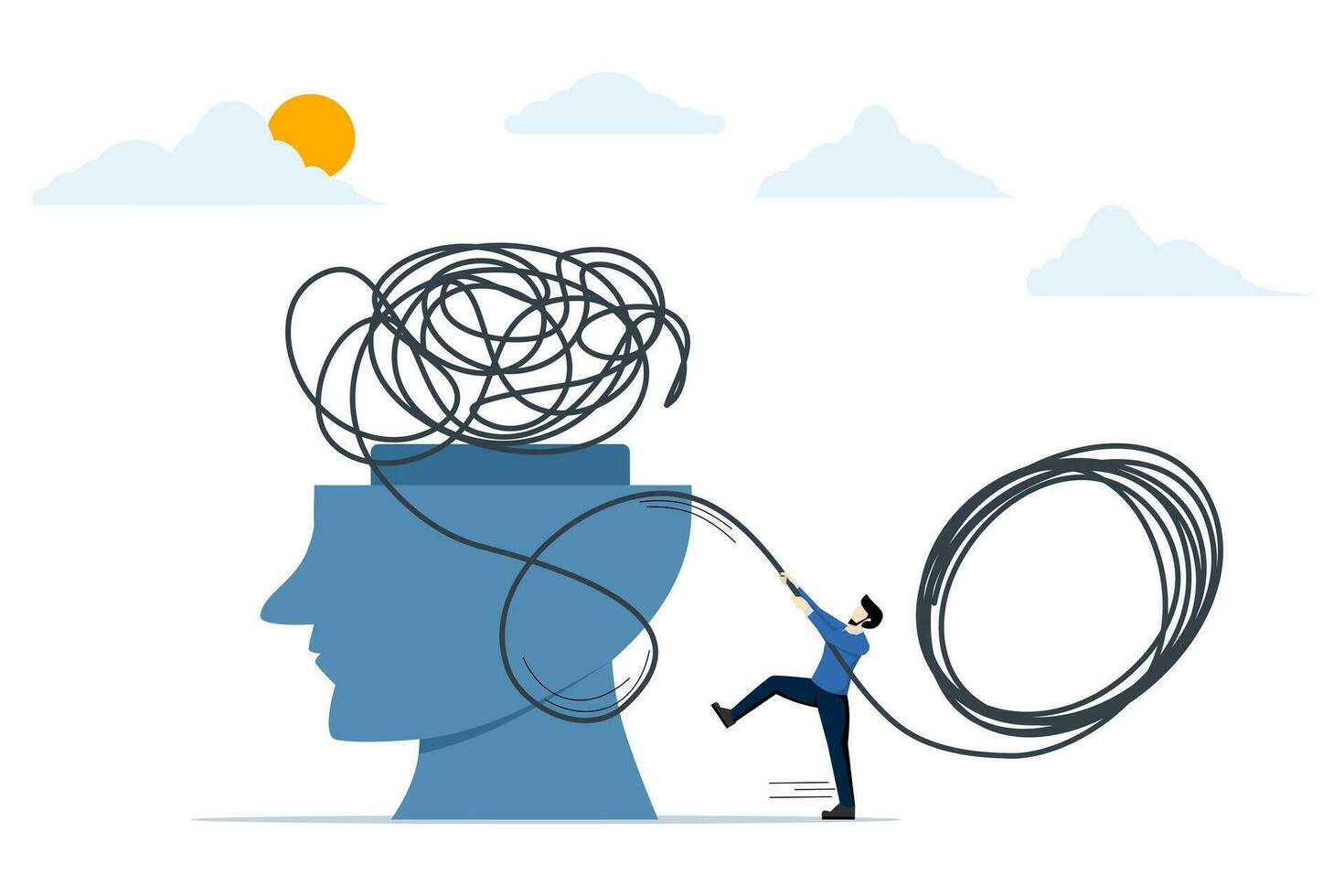The image appears to be a detailed, hand-drawn or digitally created piece set against a simple white background with no border. In the upper left corner, a yellow sun peers out from behind one of four similar blue clouds stretching across the top of the image. On the lower left side, a blue human head in profile has its top portion missing, revealing a tangled mess of black squiggly lines that resemble string or wire. A man, dressed in a blue shirt and black pants, stands behind the head and is actively engaged in pulling this tangled material, coiling it up like a rope. The man has brown hair, a beard, brown shoes, and is depicted in a dynamic pose with one leg lifted off the ground. The entire composition conveys a creative and slightly surreal daytime scene with vivid contrasts and intricate details.